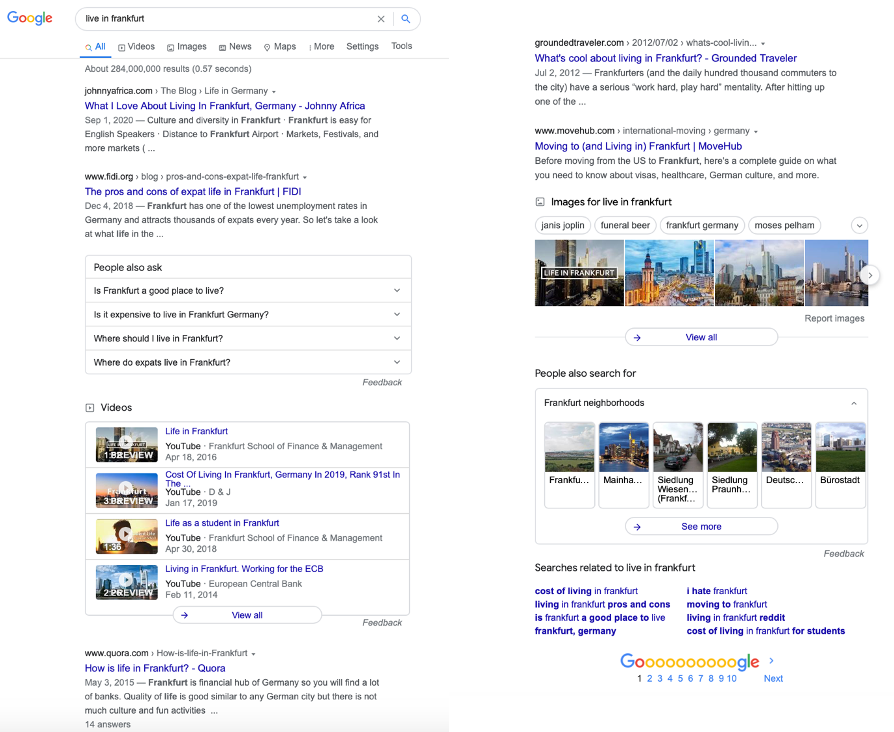The image consists of two side-by-side screenshots, likely taken from a mobile device, displaying Google search results for "Live in Frankfurt." Both screens are narrow and elongated, indicating a typical phone display.

At the top left corner of each screenshot, the recognizable Google logo is visible, alongside the search query "Live in Frankfurt." Below the search bar, the "All" section is selected, displaying a variety of search results related to living in Frankfurt.

The first result lists an article titled "What I love about living in Frankfurt, Germany" by Johnny Africa. The second result is from FIDI, discussing "The pros and cons of expat life in Frankfurt."

Between these search results, there is a "People Also Ask" box, featuring suggested questions such as:
- Is Frankfurt a good place to live?
- Is it expensive to live in Frankfurt, Germany?
- Where should I live in Frankfurt?
- How do expats live in Frankfurt?

Each question has a dropdown arrow for additional information.

Following this section, a few video links appear related to life in Frankfurt. Next, a search result from Quora asks, "How is life in Frankfurt?"

The second half of the image replicates the first half's layout on the right side. It showcases search results images labeled "Live in Frankfurt," depicting the cityscape with an option to "View All." Below these visual results, there is a "People Also Search For" section, suggesting other cities with clickable boxes. The bottom of the screens includes further search suggestions and Google page navigation links, allowing users to explore more pages of search results.